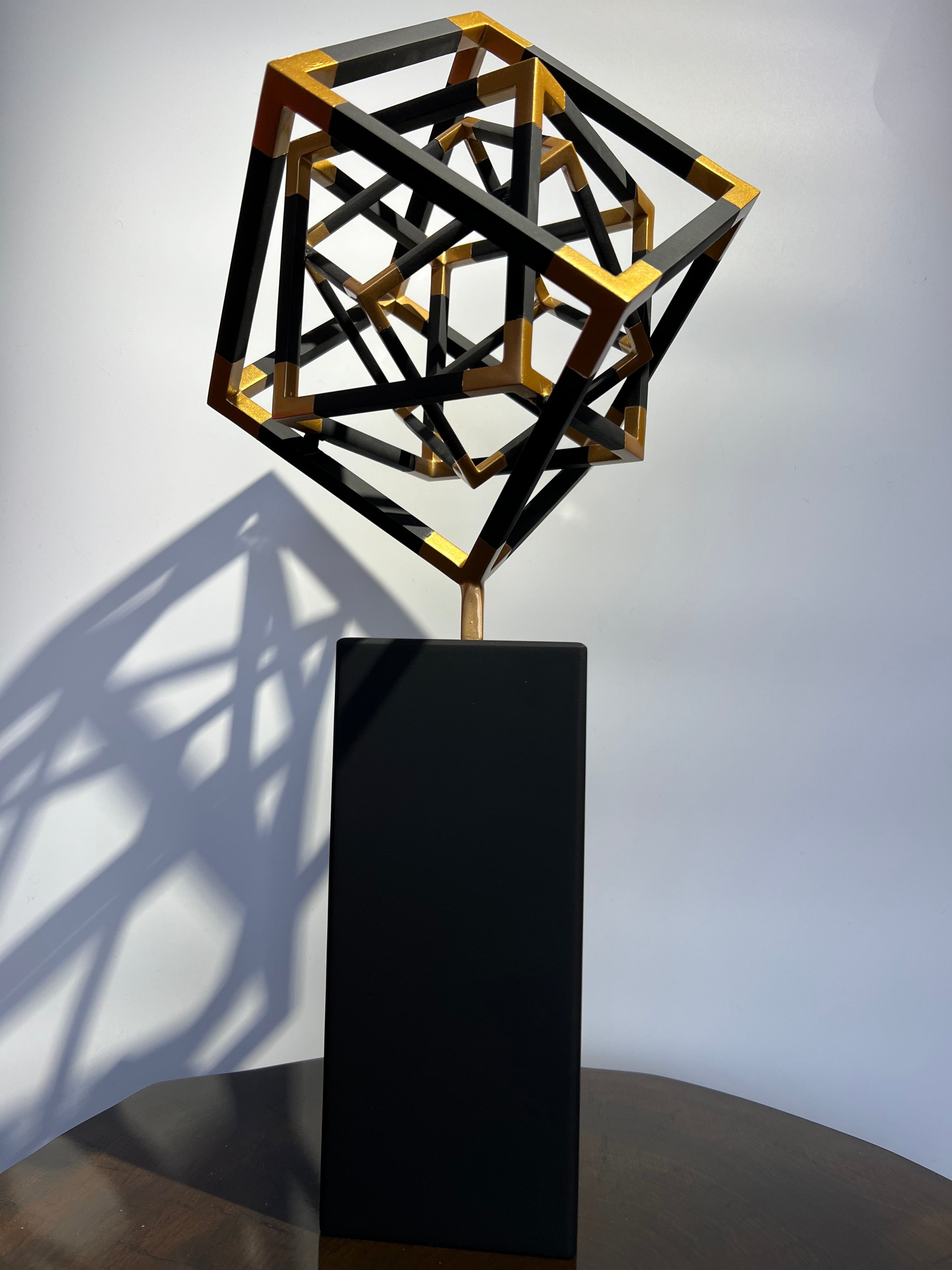The image showcases a modern art piece that resembles an award or trophy, prominently displayed on a black rectangular stand. The stand is centrally placed in the picture, though its base is not visible. Atop the stand, an artistic structure composed of three hollow cubes of descending sizes is delicately balanced. The largest black and gold cube is affixed to the stand by a slender rod, with a medium-sized cube nestled inside it, and a smaller cube enclosed within the medium one, creating an intriguing visual illusion of a square within a square within a square. The golden accents embellish the corners of the cubes, adding a luxurious touch. The background features a stark white or slightly bluish wall that sharply contrasts with the shadow cast by the cube structure. The setting suggests that this art piece is placed on a coffee table, further emphasizing the aesthetic and well-lit presentation.